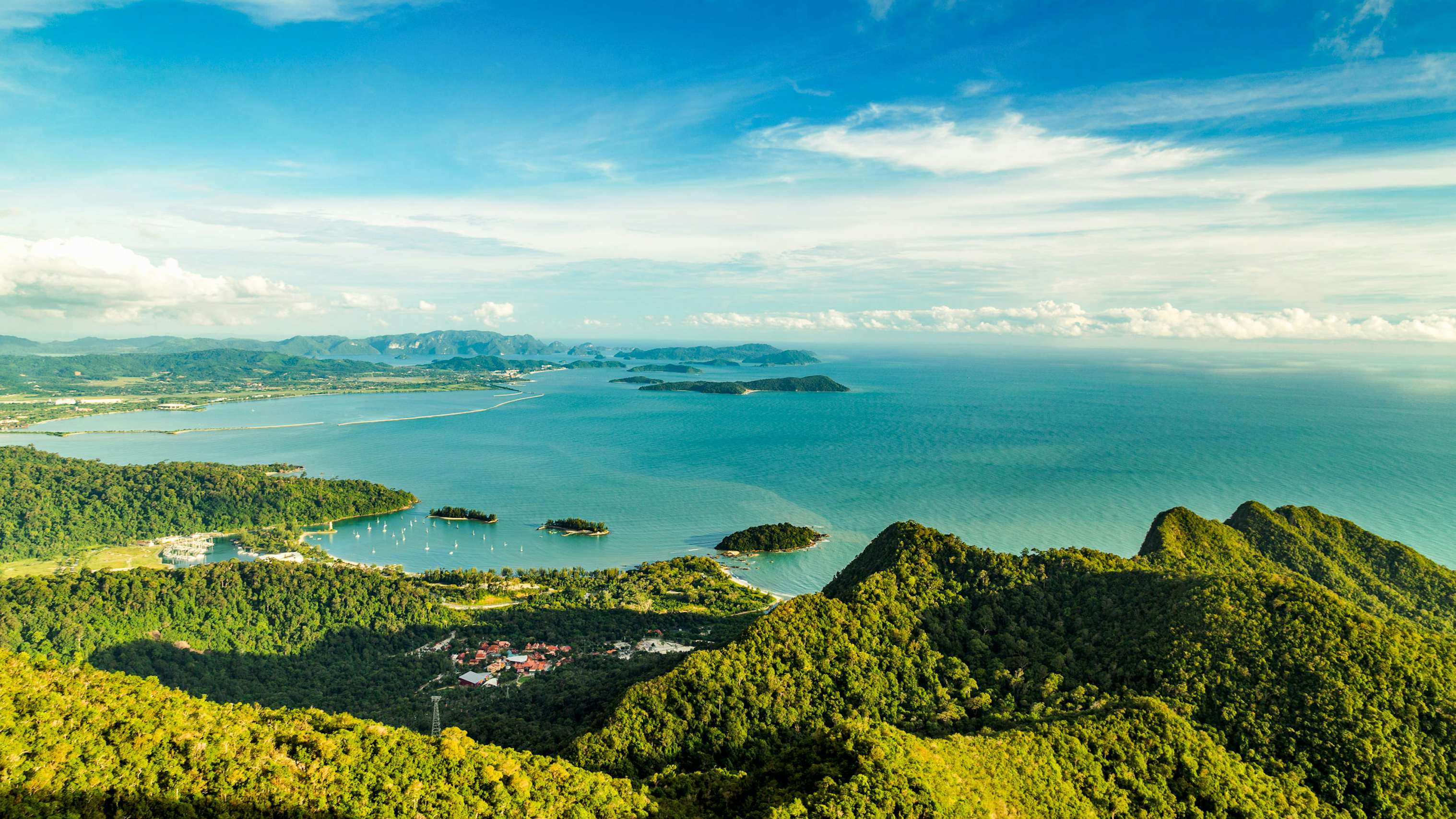An aerial landscape photo showcases a picturesque outdoor scene. At the bottom of the image, a range of lush, green mountains and hills extends from left to right, interspersed with trees and bushes tinged with yellow. Nestled within these verdant hills is a serene valley containing a small cluster of buildings with both white and orangey-red roofs. 

Beyond the mountains and valley, a vast, medium blue ocean stretches from left to right, occupying the middle of the photo. Within this expansive body of water, four small, tree-covered islands are visible near the shoreline. The distant horizon on the left is marked by another mountain range, which tapers off toward the middle, giving way to an unobstructed view where the sky seems to touch the ocean towards the right. 

The sky above is a bright blue, dotted with numerous white clouds, creating a sunny, inviting atmosphere. Additionally, scattered across the bay are tiny white specks, likely small boats, adding to the tranquil, tropical charm of the setting.